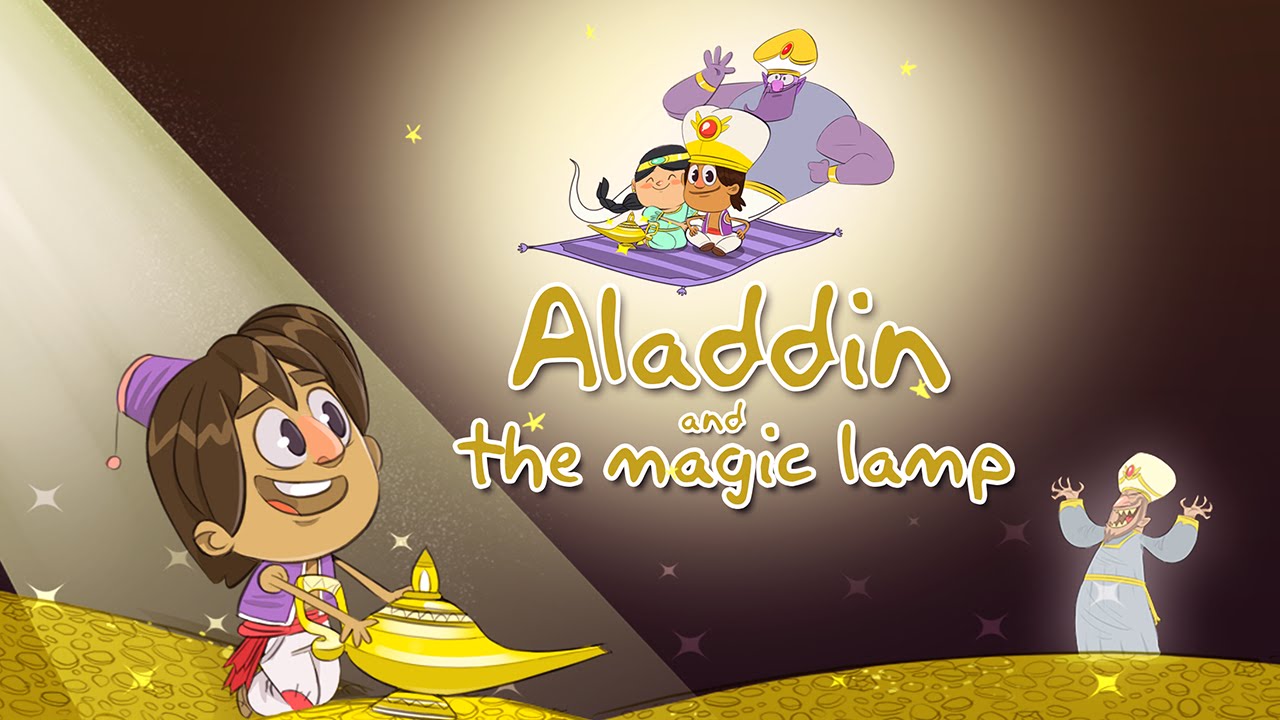The image is a detailed, computer-generated illustration titled "Aladdin and the Magic Lamp," prominently displayed in gold text outlined in white in the center. The background is predominantly silvery black with a white orb illuminating the scene. Above the text, Aladdin and Jasmine are depicted riding a purple magic carpet, with a golden genie lamp resting in front of them. Behind them, a large purple genie with a turban looms over the scene.

In the lower part of the image, Aladdin, characterized by his long brown hair, white and pink cap, purple vest, red belt, and white pants with a red patch on the knee, is seen rubbing the golden lamp while sitting on a pile of gold coins that extend from the bottom left to the bottom right. To the right, the sinister figure of Jafar is depicted in blue attire with gold accents, a white turban adorned with a red ruby, and a menacing smile. The entire scene is richly animated to portray a captivating moment from the story, illustrating both Aladdin's humble beginnings and the fantastical elements that define his adventure.